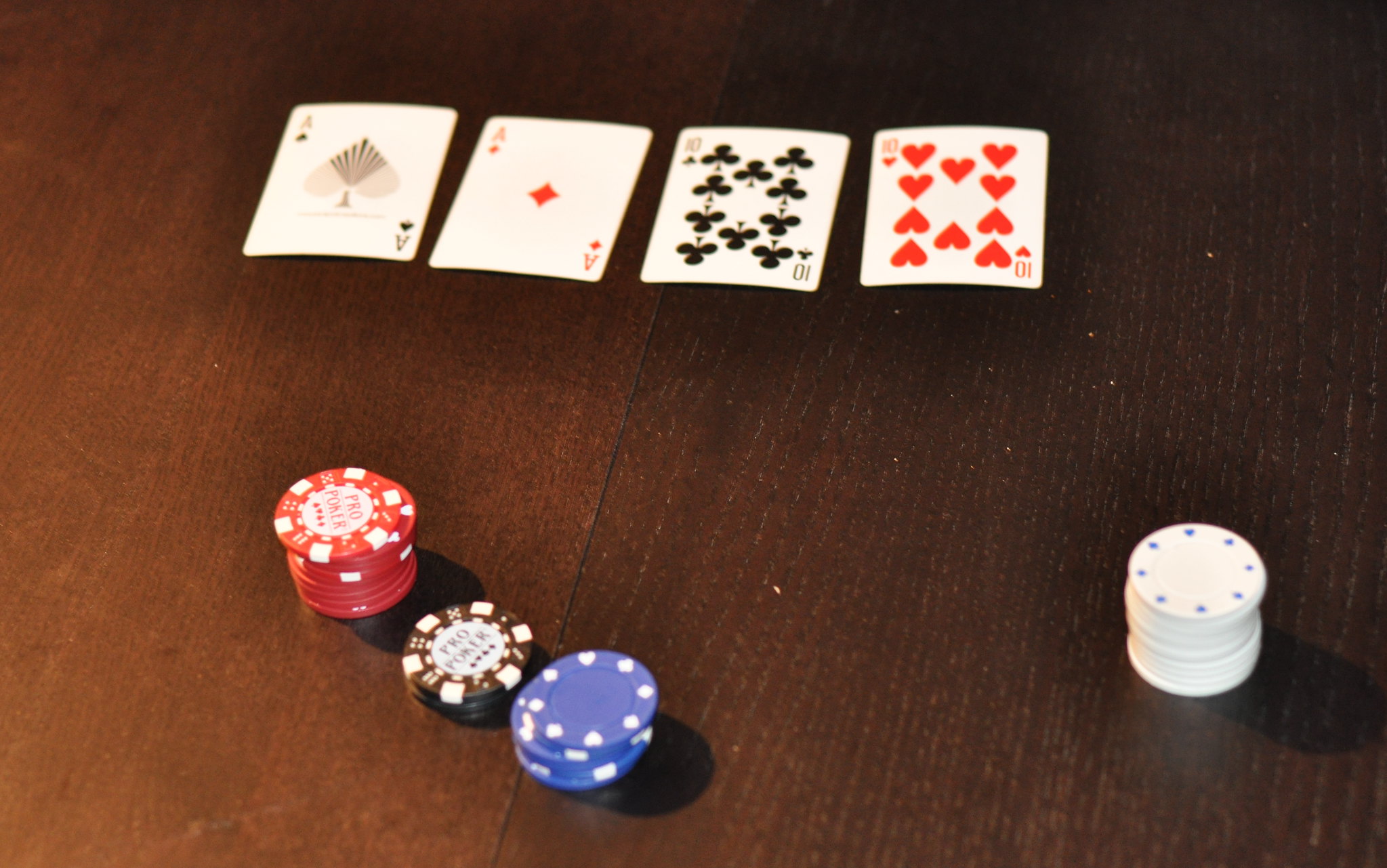On a dark brown table with visible wood grain, four playing cards are arranged horizontally across the top, slightly crooked. The first card, an Ace of Diamonds, is peculiar; in the upper left and lower right corners, the 'A' is styled as a spade. The center of the card features a faded diamond with a shadowed heart overlay, which is atypical for a standard deck. Next to this is another Ace of Diamonds, followed by a Ten of Clubs and a Ten of Hearts. The Ten of Clubs also has an unusual design, where the top left and bottom right corners display spades instead of clubs.

In the foreground, diagonally to the left, there's a stack of red poker chips. Nearby, there are four black poker chips, and slightly to the right of these is a taller stack of blue poker chips. On the far right side of the table, there is a very large stack of white poker chips.